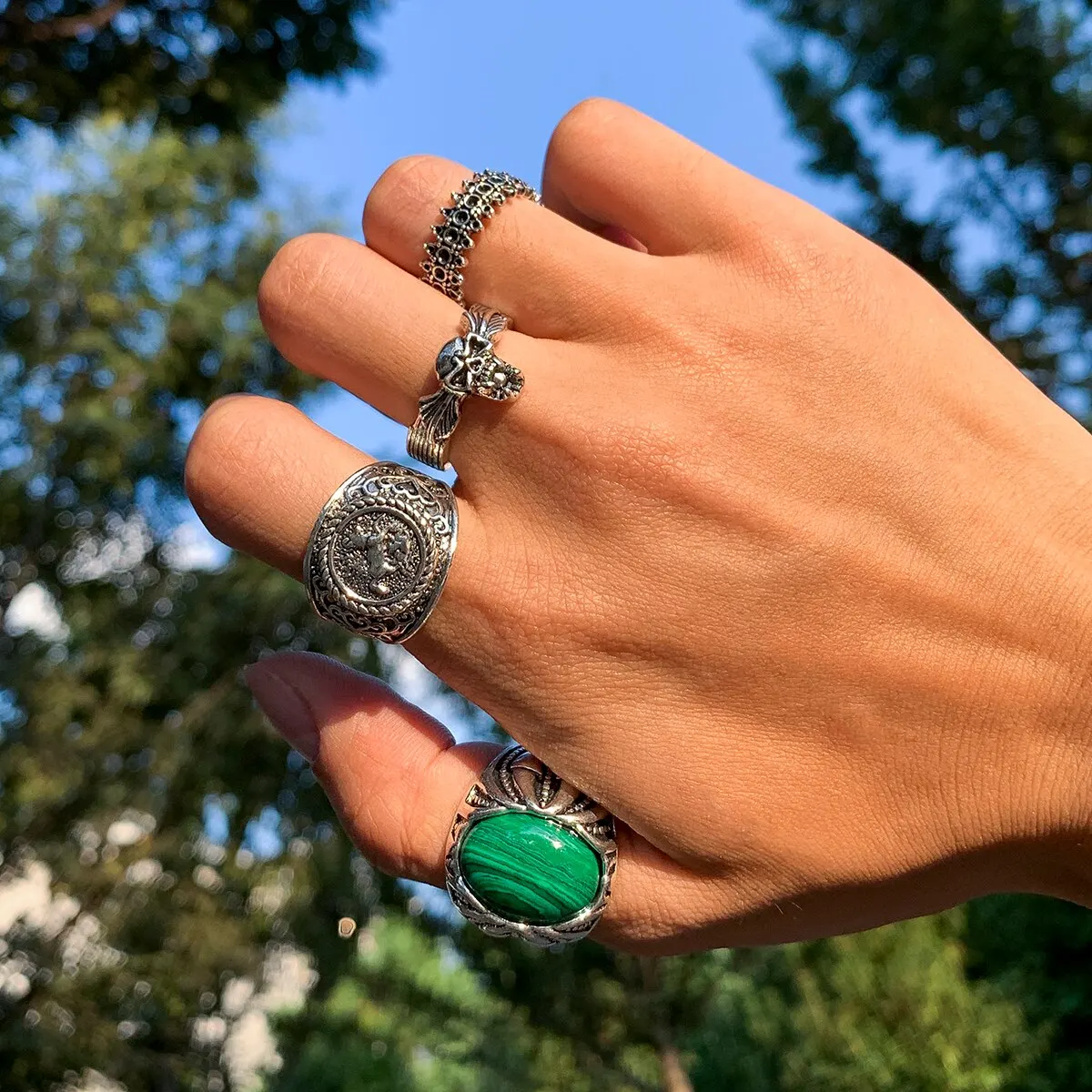The image depicts a close-up view of a person's hand, angled slightly upward and exhibiting ulnar deviation, where the fingers are bent and the palm is facing downward. The hand, which is fairly tan and suggests a lighter-skinned, likely Caucasian individual, stretches out from the right side toward the center of the image. Each finger, except for the pinky, is adorned with distinctive rings. The thumb showcases a large silver ring set with a green gemstone. The index finger bears a thick silver ring, while the middle finger features a bold silver ring with a prominent skull design. The ring finger sports a silver ring with a pattern resembling small canoes or spikes. This hand is set against a backdrop of lush green trees encircling the outer edges of the picture, primarily on the left and bottom, with the upper right corner revealing a clear blue sky.